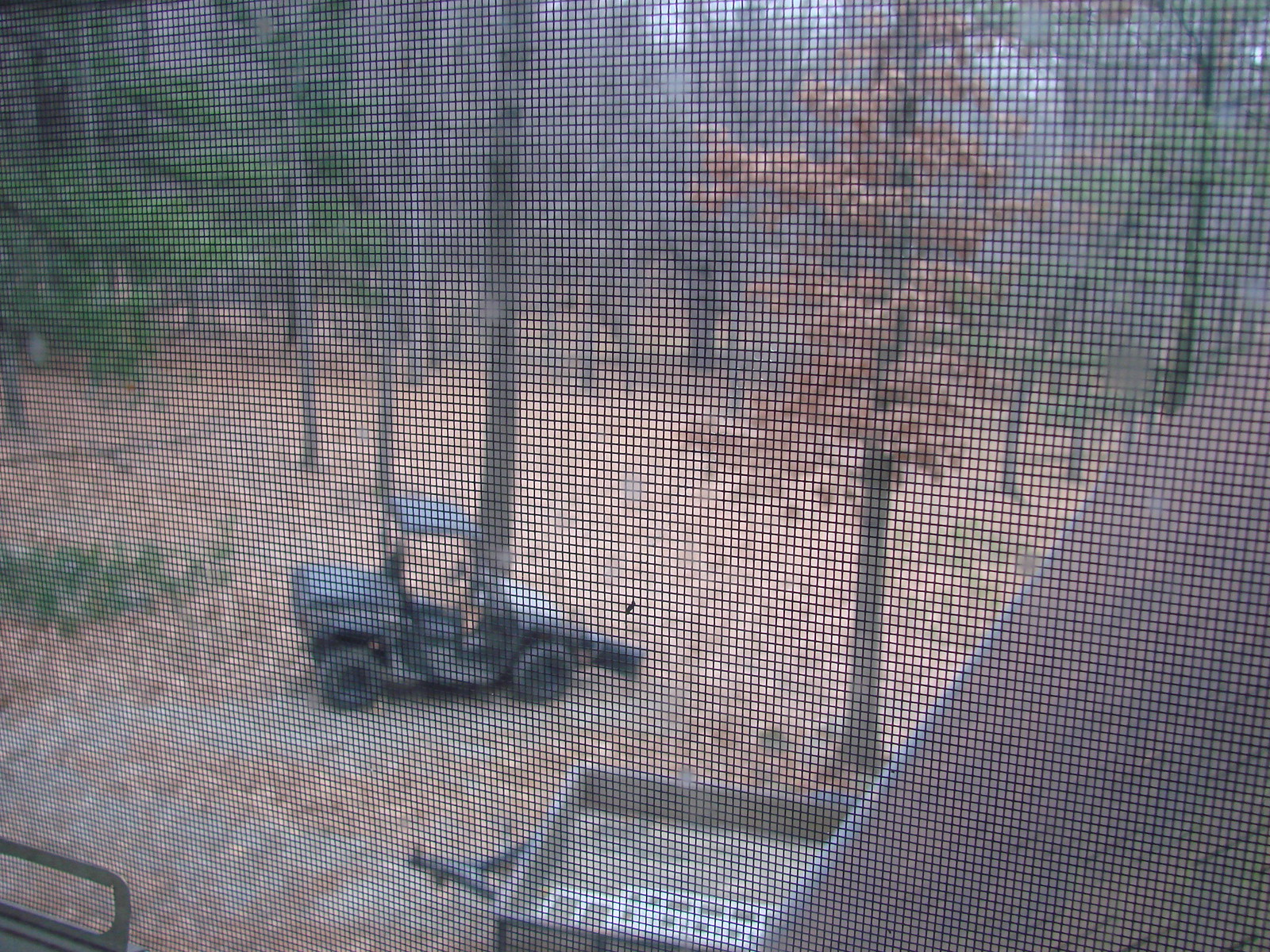This photograph, taken through a metal window screen, exhibits a significant degree of blurriness and lack of focus. The image depicts an outdoor setting marked by numerous tree trunks, most of which are slim and devoid of leafy canopy in the frame, suggesting an autumnal atmosphere with fallen leaves blanketing the ground. At the base of one of the longer, slender tree trunks, a black, two-seater open-air vehicle, possibly a golf cart, is parked and oriented towards the right. In the lower center of the image, a grill or similar outdoor appliance can be faintly discerned. Additionally, a white triangular shape is visible in the lower right corner, though its nature and connection to the scene remain unclear.